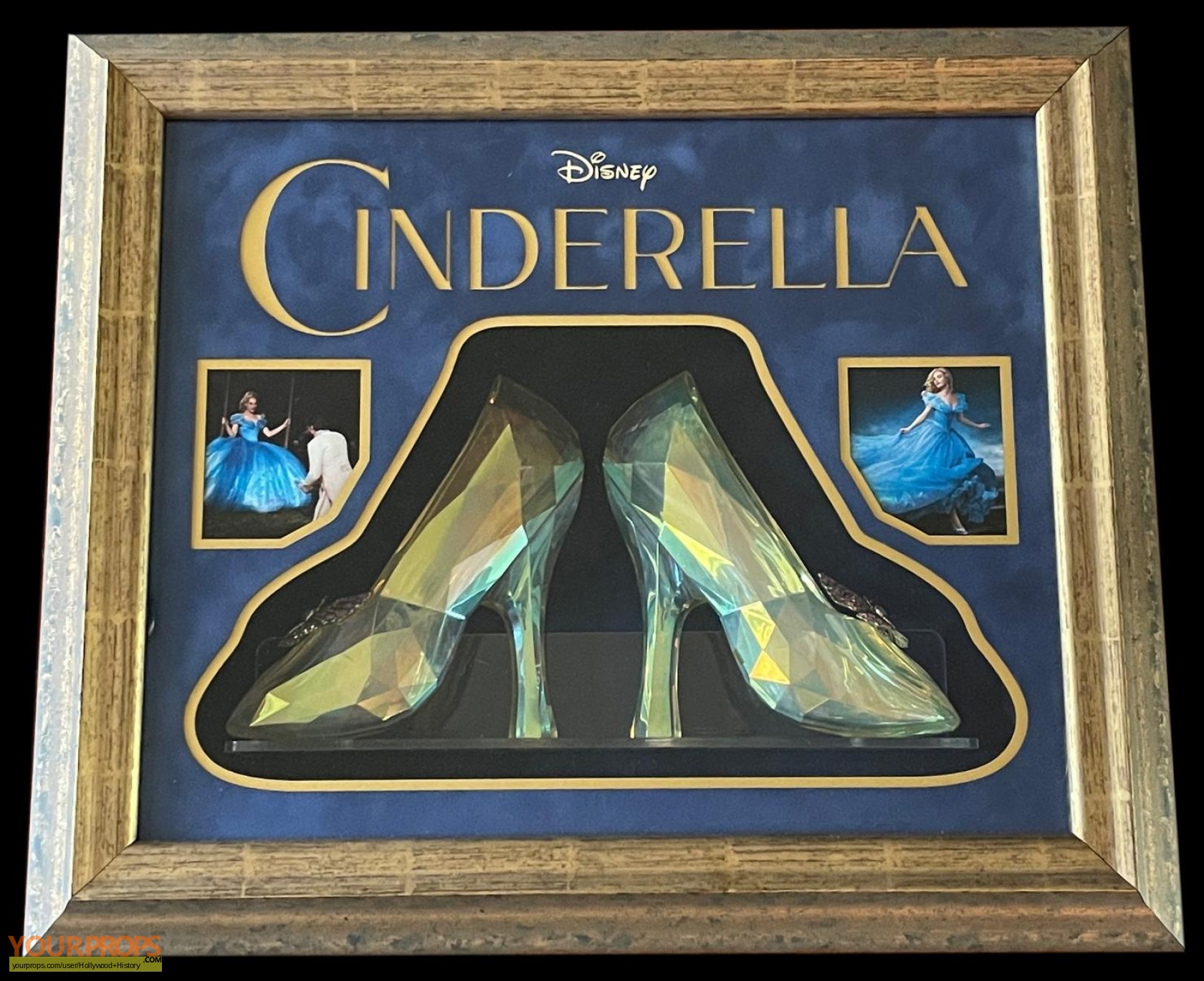The image features a medium brown wooden rectangular frame encasing a keepsake of Disney's Cinderella. The background is a striking dark blue with a mottled pattern. At the top, in small gold letters, it reads "Disney," and below it, in prominent big gold letters, it says "Cinderella." Central to the display are two crystal slippers resting on a lucite shelf, each with delicate butterfly accents and a subtle gold reflection. To the left, there's an image of Cinderella in a blue dress with the prince kneeling and fitting the glass slipper on her foot. To the right, another image shows Cinderella in her blue gown, running away and losing her slipper. The overall presentation highlights the iconic elements of the Cinderella story, capturing its magical essence.